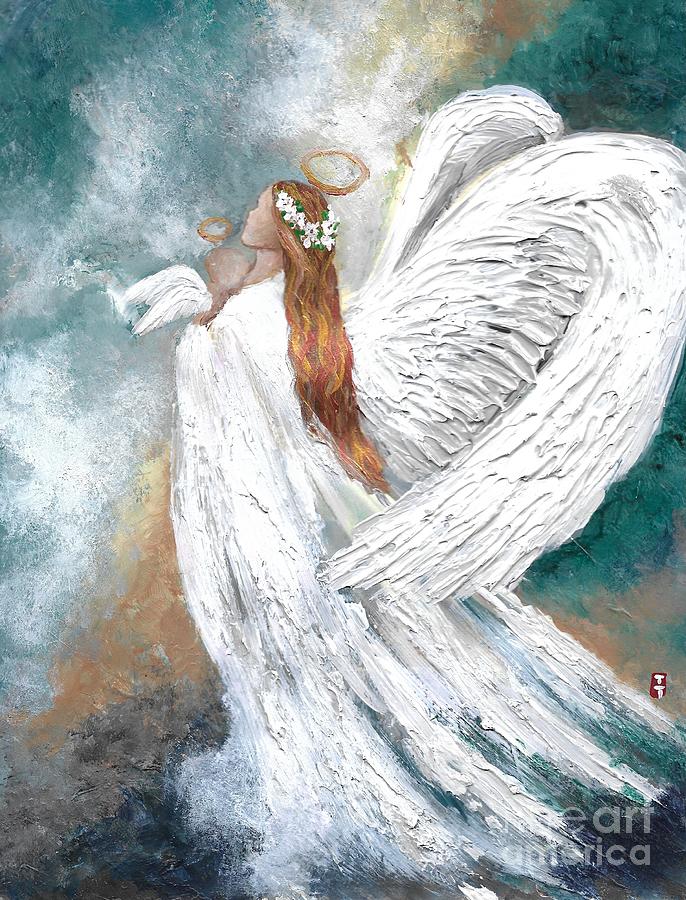The painting depicts a serene, angelic figure positioned centrally, characterized by her long, flowing orange-red hair that cascades down her back, almost reaching her waist. She is clad in an elegant, white dress with prominent, large white wings extending behind her. The angel is looking upwards toward the sky, her expression hidden as her face appears featureless. Above her head hovers a light brown halo, emphasizing her divine nature.

The background is a gradient of blue-green or teal, which becomes darker near the bottom of the image, adding depth and contrast to her white attire and wings. Nestled in her arms, she cradles a smaller angel, identifiable by its miniature wings that reach up to her neck. The rough, textured edges of the painting add a tactile element, making the brushstrokes visibly stand out.

To the right of the angel, near the edge, sits a small orange box containing the initials "T.T." Additionally, in the lower right corner, there's an inscription reading "the art America," which could indicate a signature or a label associated with the artwork.